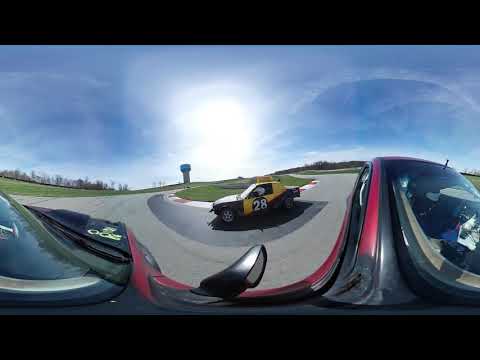The image depicts a dynamic racetrack scene featuring multiple race cars captured with a fisheye lens that distorts and skews the perspective. In the foreground, from the viewpoint of a red and black race car, the viewer's eyes are drawn to a prominently positioned yellow and black two-door race car bearing the number 28 in white text inside a black circle on its side. The yellow car, with a mostly yellow body and black hood, is driven by a person wearing a white helmet. The racetrack, made of gray asphalt, is bordered by grassy infields and outfields, with red and white boundary markers along the curve of the track. In the distance, the landscape includes a forested area and a water tower on the horizon under a clear blue sky with the sun visibly centered. The fisheye lens effect causes elements of the red race car from which the photo is taken to appear curved and abstract, particularly noticeable in the black wing mirror and the U-shaped body extending across the sides of the image.